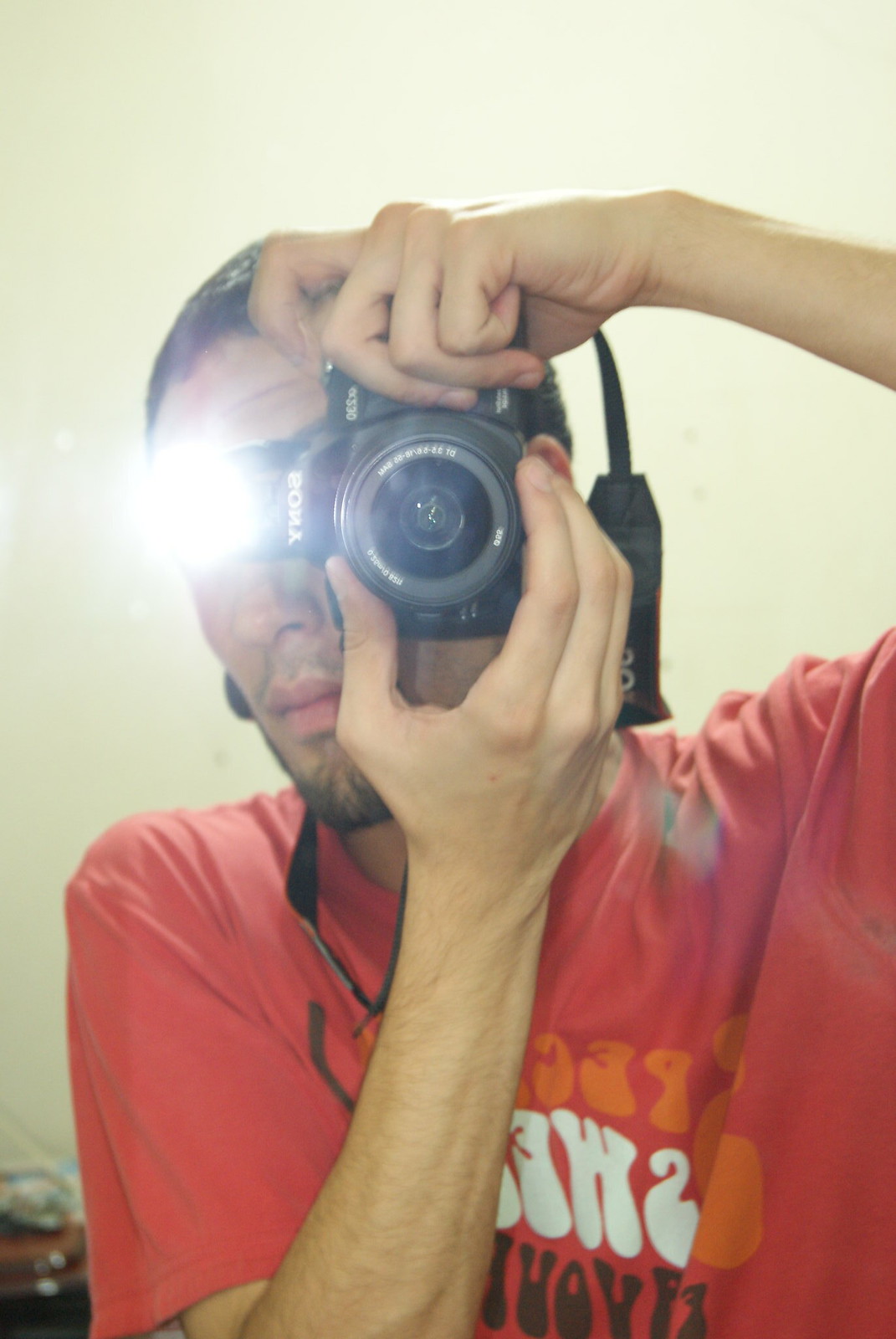The image captures a man taking a mirror selfie with a Sony DSLR camera. He holds the camera vertically, covering his right eye while his left eye is obscured by the flash, creating a bright white light over his face. His hands are firmly clasped around the camera, with one on the adjustment wheel. The man has short, dark hair, a mustache, and a stubbly beard. He is wearing a red T-shirt adorned with text in orange, white, and black, though the specific words are indiscernible due to the mirror reflection. The background features a green hue with a white wall and indistinct objects blurred on the floor. The overall color palette includes the red of the shirt and the reflected colors of the letters. The photo also includes light streaks, adding to the dynamic and somewhat gritty aesthetic.